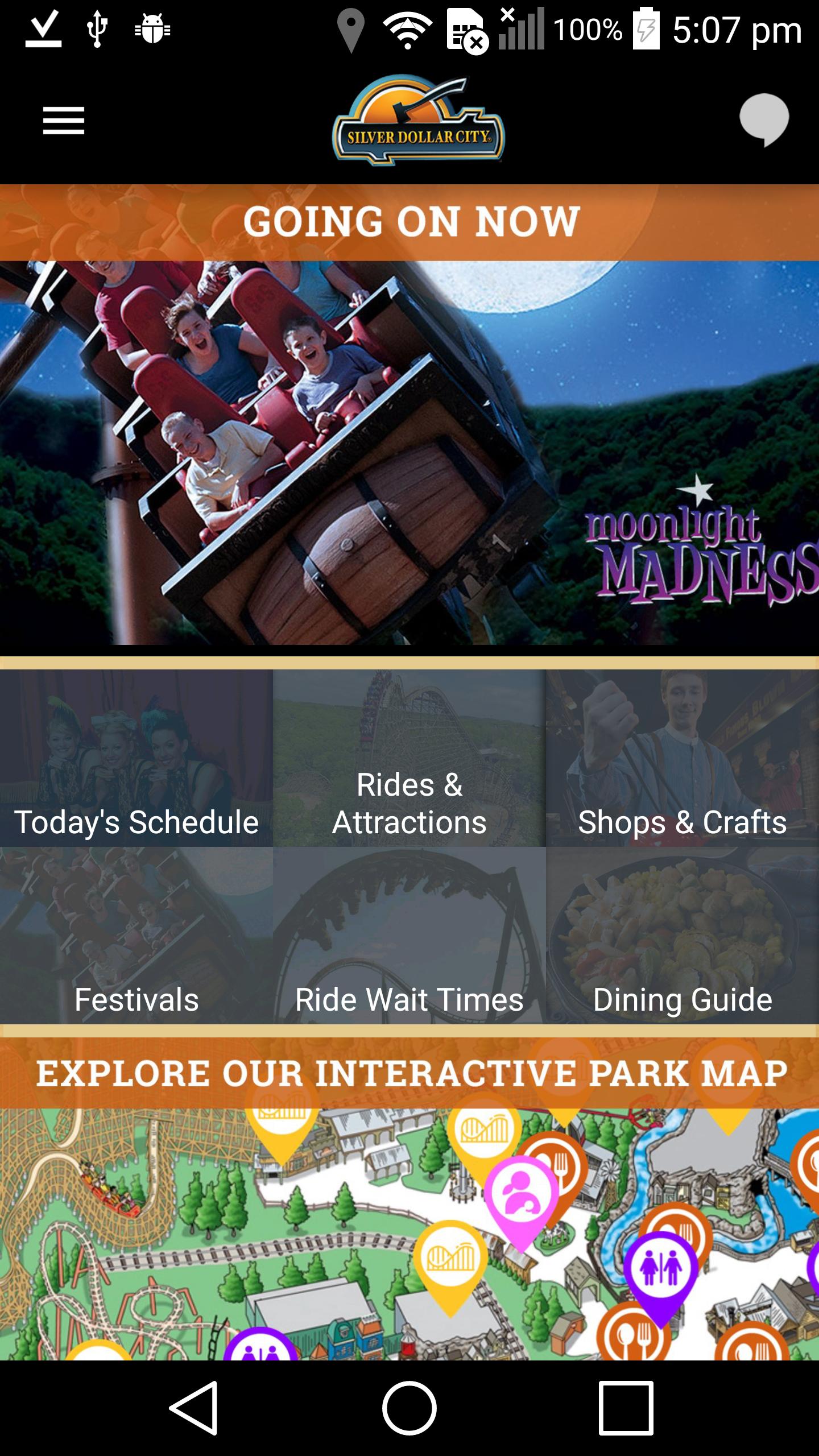Visible at the top of the screenshot is an emblem that reads "Shafter Dollar City," with a sun icon partially obscured by a black stripe. Superimposed over the sun is an axe, creating a striking image. Just below this emblem, a brown bar spans the width of the image, featuring the text "Going On Now" in white.

In the main part of the image, there's a lively photograph of people riding a rollercoaster. The front car of the rollercoaster is designed to resemble a brown barrel. The riders are captured mid-experience, laughing and screaming with excitement. The backdrop features a vibrant blue sky, a visible moon, and lush green trees, enhancing the atmosphere of thrill and adventure. 

Across the image, in bold purple lettering, the phrase "Moonlight Madness" stands out, indicating a special event or ride theme. The rollercoaster car is shown dramatically tilting to the side as it speeds along the track.

Below the main image, the screen transitions to a section displaying the day's schedule, listing various categories like rides, attractions, shops, crafts, festivals, ride wait times, dining, and guide. A colorful, cartoonish map of the entire park is also included, inviting visitors to "Explore Our Interactive Park Map."